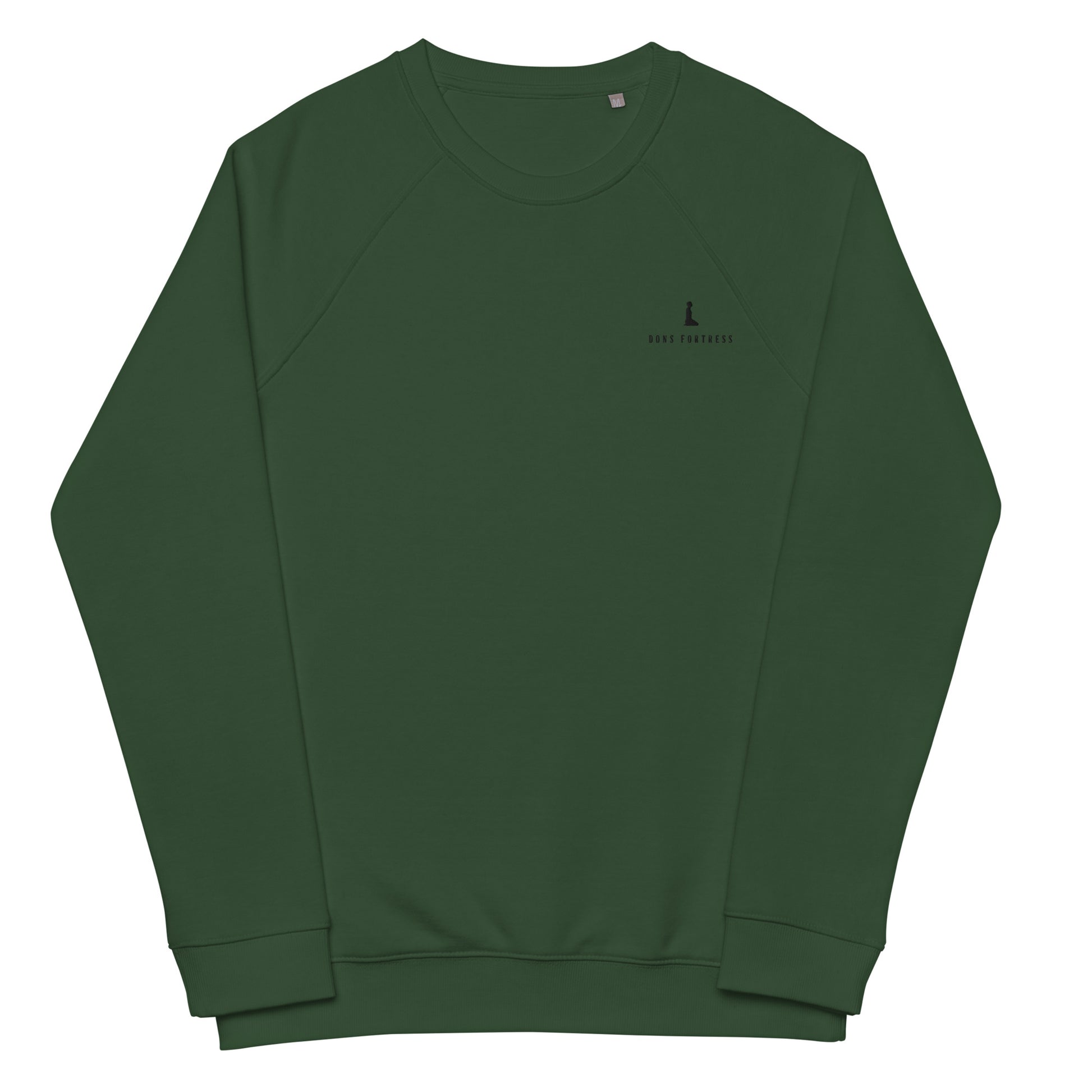In the image, a men's sweater is displayed on a white surface, showcasing its sophisticated design and rich forest green color. The sweater exudes simplicity and elegance, with a classic, dark green hue that is both versatile and timeless. It appears to be either a large or extra-large size, providing a comfortable and relaxed fit. The sleeves are neatly folded inward, adding a touch of precision to the presentation.

On the right side of the chest, there is a subtle designer logo. This logo is relatively small and difficult to make out, resembling a black lighthouse accompanied by some lettering beneath it. Additionally, the sweater features a small neck tag located on the right side of the back neck area. This tag is a small white square, adding a minimalistic detail to the overall design. The clean and well-structured layout of the sweater against the white background enhances its classic appeal.